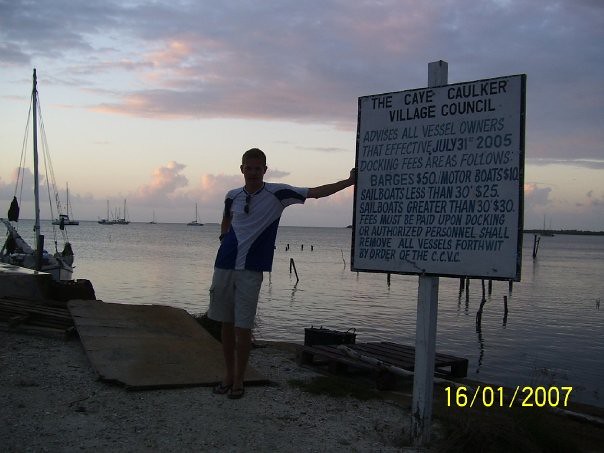The photograph captures a young man standing near the coast of what appears to be an ocean, with sailboats dotting the water in the background. The sky is an intriguing blend of purplish, pinkish, white, and gray hues, suggesting the approach of evening. The man, centrally positioned in the image, leans against a white sign marked with black and green text. The sign, which belongs to the Cave Caulker Village Council, advises vessel owners about docking fees effective from July 31st, 2005, detailing charges for barges, motorboats, and sailboats of various sizes. The man is casually dressed in white shorts, a blue and white t-shirt, and sunglasses, standing on a gravelly shoreline. A yellow time stamp at the bottom right corner of the image reads '16-01-2007'.